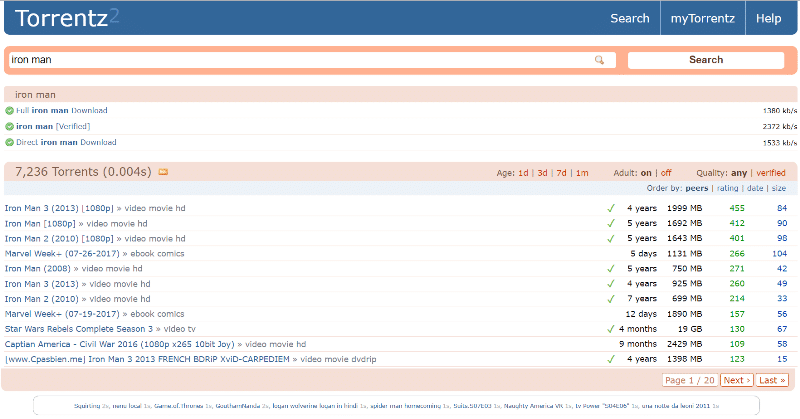This screenshot depicts the homepage of the defunct torrent search engine, torrents2.com, which has undergone various rebrandings such as torrents2.org and torrents2.az over its lifespan. The website is no longer officially online; this appears to be a replicated version of its interface, likely operated by third parties and laden with malware, making it untrustworthy.

At the top of the page, there is a prominent search bar displaying the query "Iron Man." Below the search bar, search results indicate that there are 7,236 torrent files found for "Iron Man." The subsequent listings feature various downloadable torrents primarily for different versions of the Iron Man films. For example, prominently displayed among them is "Iron Man 3 (2013) in 1080p," categorized under video movies in high definition (HD). The list on this single page features nearly a dozen different download options, showcasing the breadth of content once provided by this now-defunct search engine.